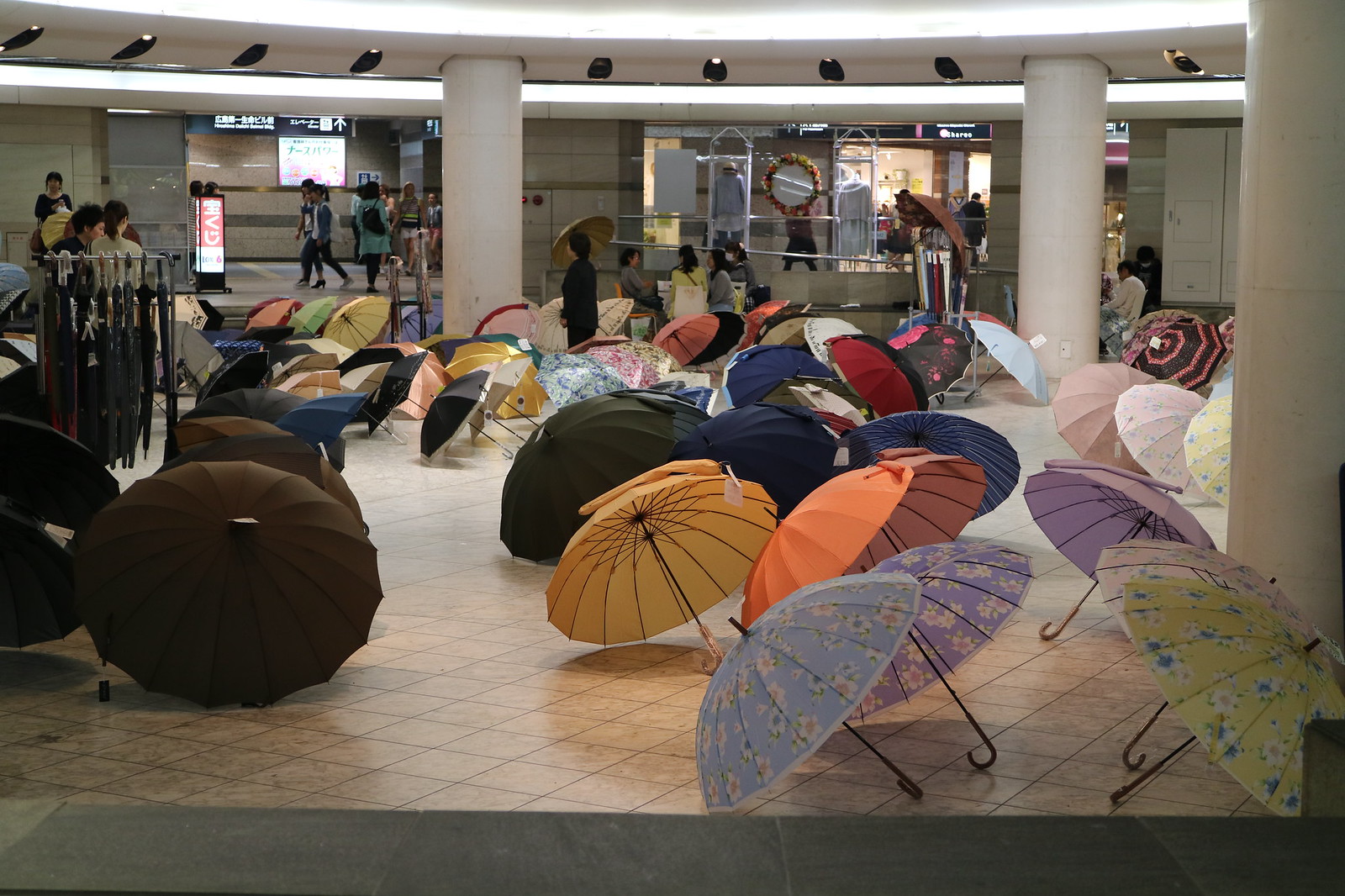This indoor color photograph, taking place in what appears to be a spacious area within a mall or possibly an airport, showcases an art exhibition or a unique retail display featuring a striking array of approximately 100 decorative umbrellas. The scene is anchored by beige tile or marble flooring and is punctuated by large, white support columns—three of which are prominently positioned. The photograph is well-lit, with white fluorescent lighting illuminating the space, ensuring every detail is captured sharply.

The foreground and background are dominated by opened umbrellas, some regular black ones and others boasting a vibrant palette of colors, including yellow, pink, peach, blue, orange, purple, and red. These umbrellas feature a variety of patterns like spirals and floral prints, offering a visually arresting contrast against the neutral flooring. A small rack on the left side of the image holds folded umbrellas, indicative of them being on display, potentially for sale.

People can be seen walking in the background, adding liveliness to the scene, and a row of glass-fronted stores lines the back wall of this open space. Additional details, such as a few vending machine signs and a small table for resting, populate the periphery of the photograph. Some signs appear in Asian characters, suggesting the location could be somewhere in Asia. Overall, this detailed and well-lit image beautifully captures the intricate arrangement of umbrellas amidst the bustling environment of a mall or airport setting.